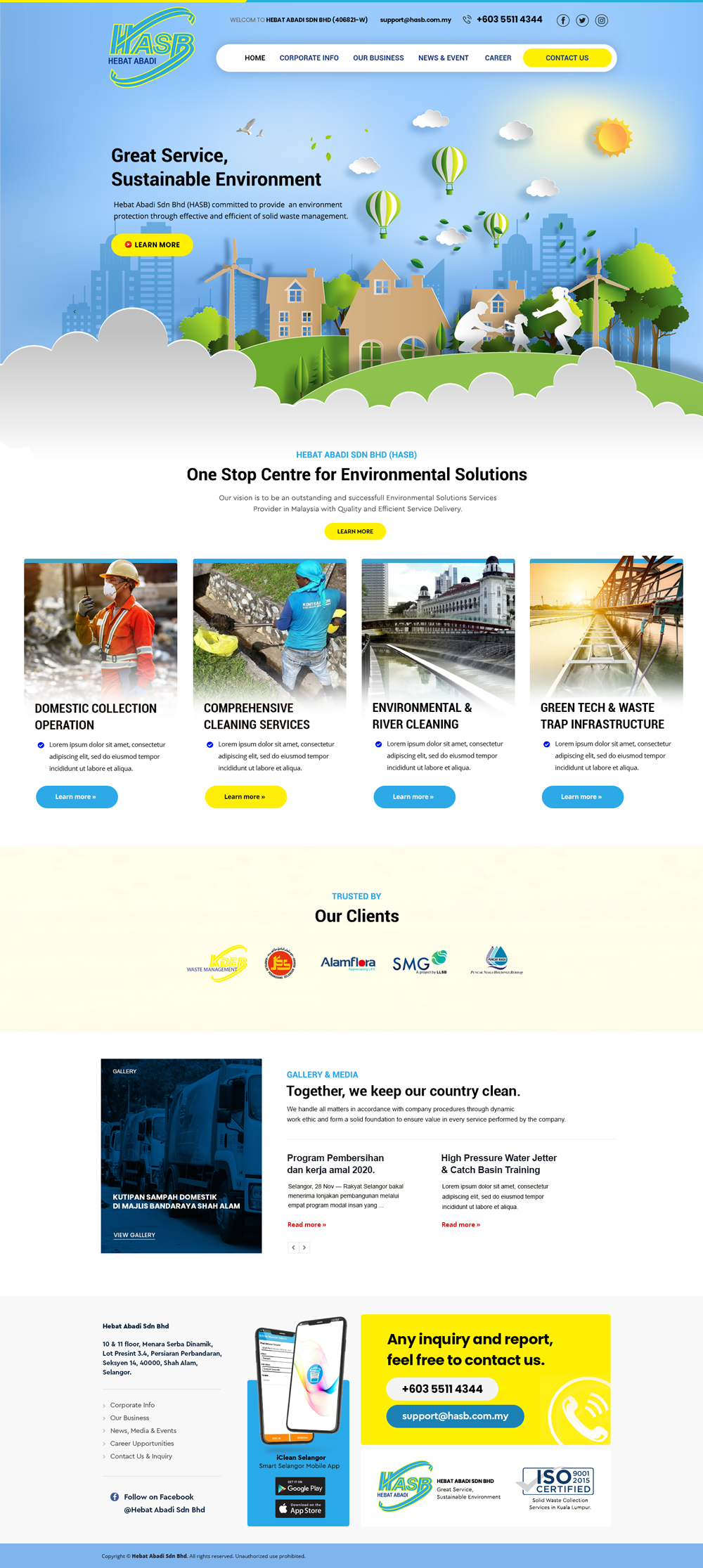The image is a vertically-oriented rectangle, captured from a mobile app or website. At the very bottom, a thin blue border contains some writing, although the font is so small that it's unreadable. Starting from the top of the image, the background features a cartoonish cityscape with a bright blue sky and a drawn sun positioned on the right side. The scene includes a playful family, illustrated in white, frolicking on a green hill. Surrounding them are several drawn elements: trees, houses, fluffy clouds, balloons floating in the air, and darker blue buildings in the distant background.

Embedded within the cloud imagery is the text "Great service, sustainable environment." Directly beneath this statement, there's a paragraph of text that is too small to read, accompanied by a yellow oblong box with black writing that says "Learn more." Near the top of the image, a horizontal menu is displayed within a white oblong circle. The menu items include "Home" on the left side and a yellow box labeled "Contact Us" on the right.